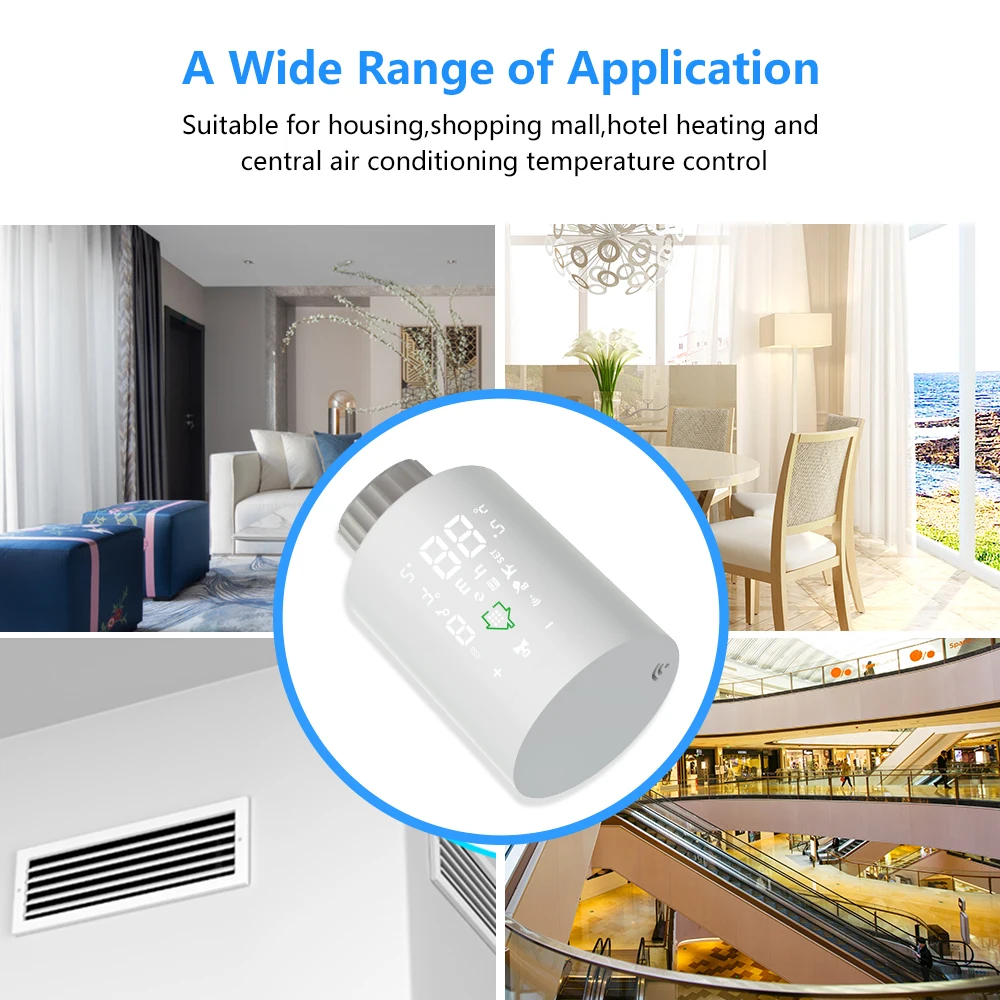The advertisement prominently features the text "A Wide Range of Application," in light blue at the top, and "Suitable for housing, shopping mall, hotel, heating and central air conditioning temperature control" in black below it. At the center is a white circle with a light blue border, showcasing a smart cylindrical temperature control device with digital numbers displaying '88' and icons such as a green outline of a home and a Wi-Fi symbol. The layout around the device is divided into four quadrants showing applications for different settings. The top left quadrant features a hotel room with a white couch and two navy ottomans. The top right quadrant displays a dining room filled with cream, beige, and white tones, complete with a dining table and chairs set by a window. The bottom left quadrant displays a wall with a ventilation system or air return vent, while the bottom right quadrant shows the inside of a brightly lit shopping mall with an escalator and people shopping. The overall presentation is in vibrant, clear color, emphasizing the wide range of environments suitable for the device’s use.